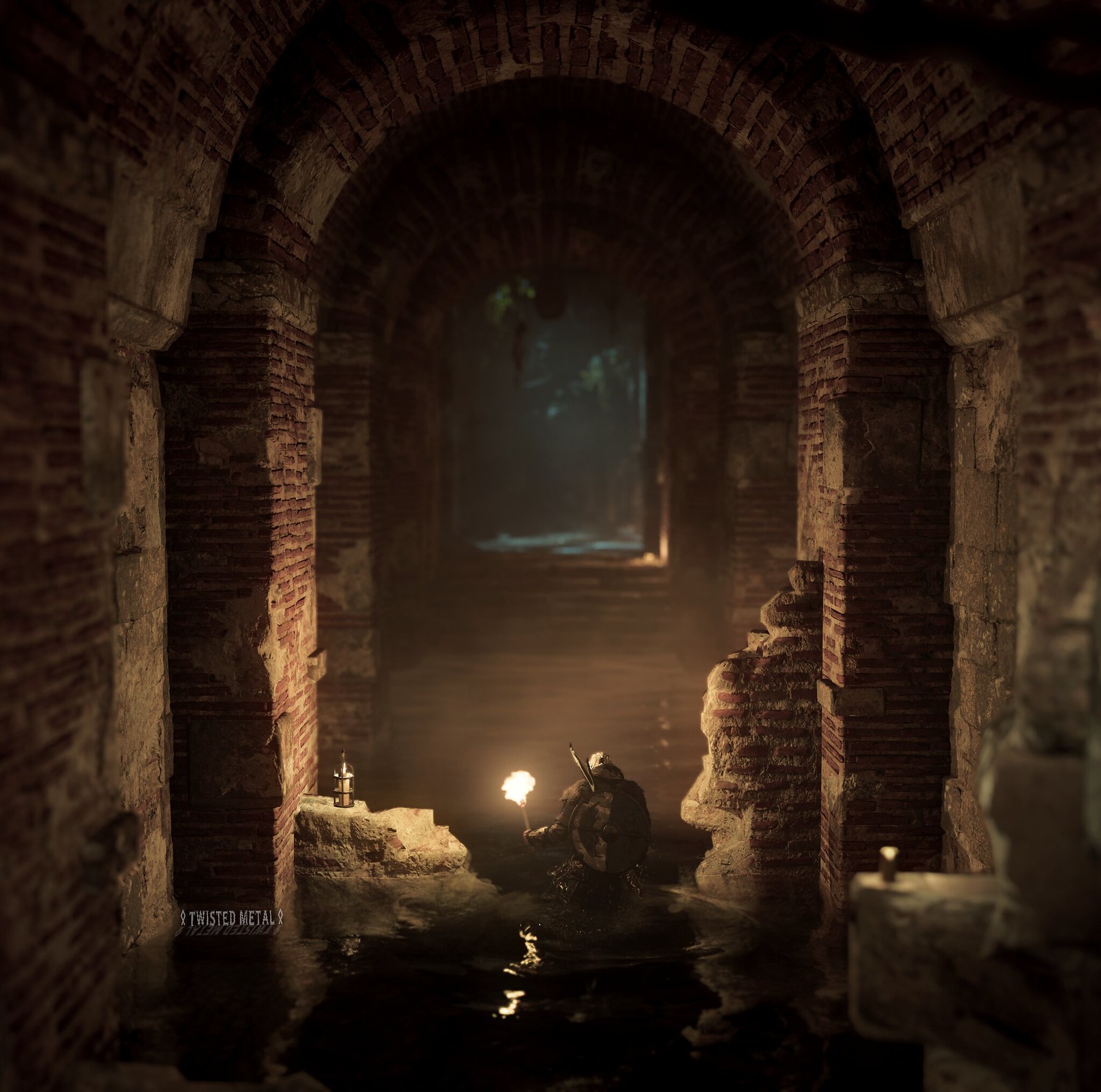The image depicts a scene from a highly realistic modern video game. It shows a character, whose back is turned to the viewer, waist-deep in water within an arched, brick-walled underground passage resembling a sewer or dungeon. The dark environment is punctuated only by the light from the torch held in the character's left hand, casting glimmers on the water's surface and faintly illuminating the red brick and gray mortar walls. The character appears to be clad in dark-colored armor and has a round shield attached to their back, potentially indicating a soldier or warrior. The lower left corner of the image has faint white text reading "Twisted Metal," suggesting either the game's title or a thematic alignment with heavy metal aesthetics.